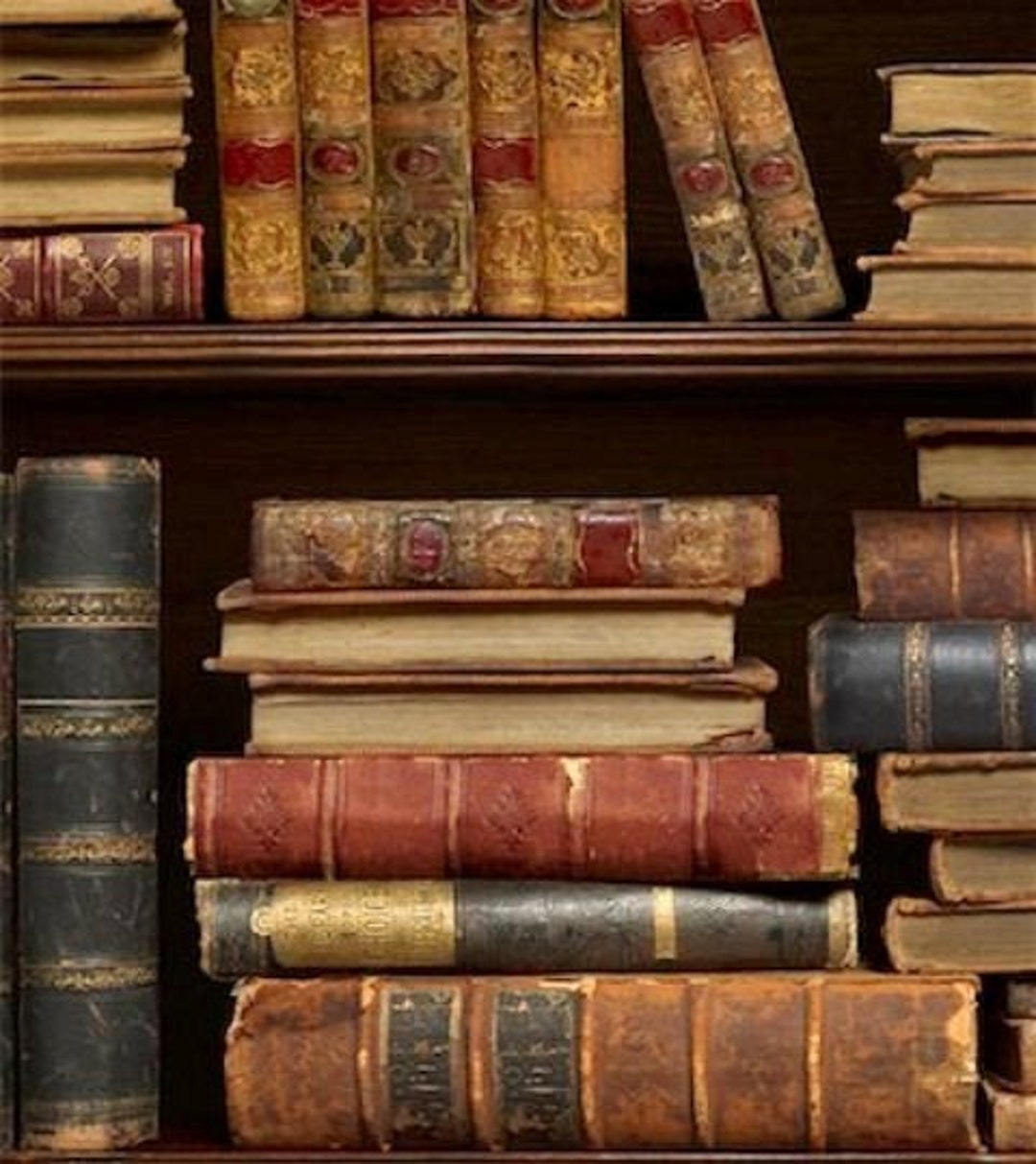This is a detailed photograph of two shelves on a dark brown wooden bookcase filled with very old, antique books. 

**Top Shelf:**
The top shelf is partially cut off at the top of the frame but clearly shows books arranged in three distinct sections. At the left and right ends of the shelf, there are stacks of four books each laid flat. These books appear aged, with no visible writing, and are in shades of yellow, red, and black. In the middle, seven upright books with their spines facing outward showcase intricate patterns in light brown and light green with red lines across them. These upright books are flanked by flat stacks, leaning slightly for support.

**Bottom Shelf:**
The bottom shelf is fully visible and holds several books arranged both upright and in stacks. On the far left, a large, mostly black book with some golden colors and trim stands vertically. Toward the center, there is a meticulously stacked pile of six books, the largest and thickest at the bottom, tapering to the smallest and thinnest at the top. The bottom three books in this stack present their spines outward, showing varied dark brown, black, and red colors, while the top books show their pages. To the right, there's another stack comprising eight to nine books, continuing the theme of aged and antique volumes. 

The overall impression of the bookshelf is one of historical value, with all the books presenting an antique, intricately designed aesthetic.